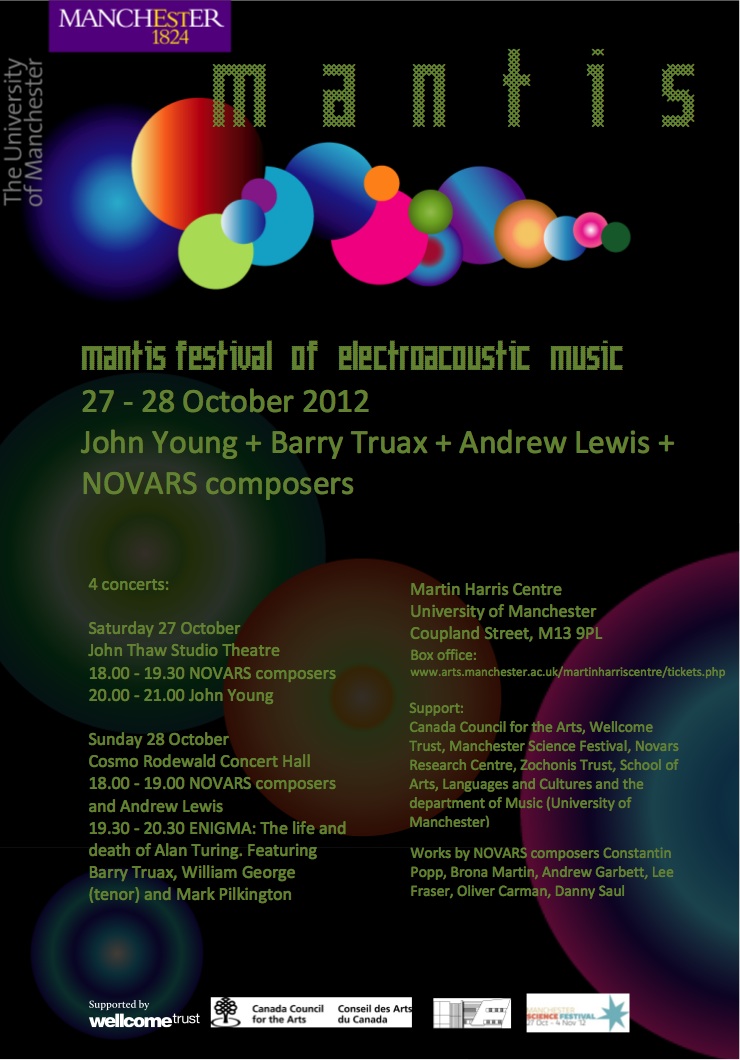This image prominently features the title "Manchester, 1824" situated at the upper left-hand corner in a notable font style. Adjacent to this, and aligned vertically, is the text "The University of Manchester," with "The University" positioned slightly higher and "Manchester" directly below. This text is relatively smaller and located in the bottom left corner of the "Manchester, 1824" header.

The primary background of the image is a sleek black, adorned with vibrant, multicolored bubbles scattered throughout. Positioned at the center top of the image, the word "Mantis" is displayed in a green, pixelated font. Below this, a horizontal arrangement of bubbles adds a dynamic visual element to the design.

Further down, the text "Mantis Festival of Electroacoustic Music, 27-28 October 2012" is centrally placed, followed by the names of featured performers: John Young, Barry Trowe, Andrew Lewis, and Norvis Composers. The lower section of the image contains two columns detailing a schedule of four concerts. Each element is meticulously arranged to promote the Mantis Festival in a visually engaging and informative manner.